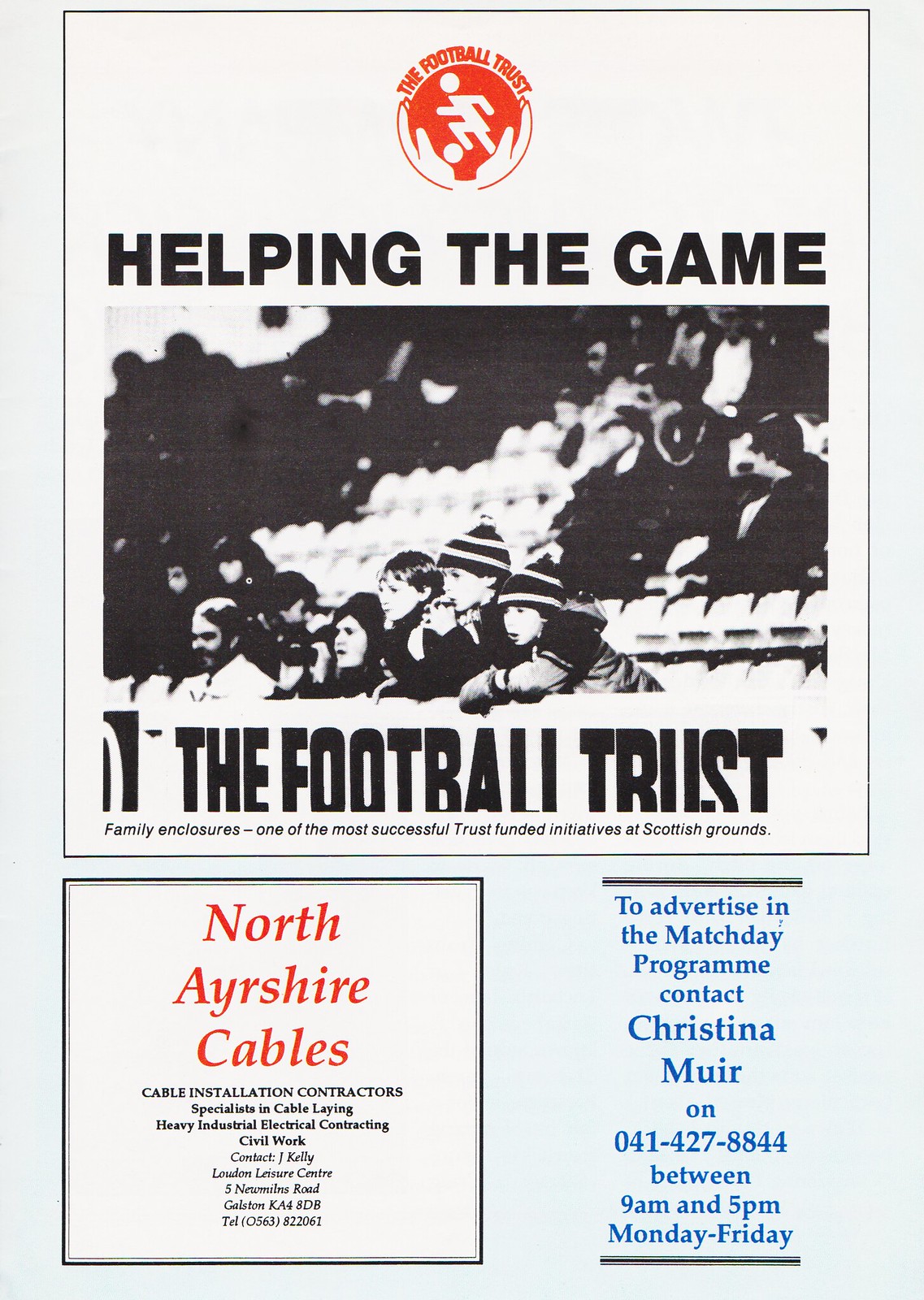At the top of this scanned magazine page, there is a prominent circular logo with a red ball containing a silhouette of a soccer player kicking a white ball towards the left. Above the logo, it reads "The Football Trust," and below it, two white hands are seen holding the red ball. Directly beneath this, in bold black letters, the text states "Helping the Game." Further down, a black and white photograph depicts several children in winter hats in the spectator area, intently watching a football match. In front of them, a banner prominently displays "The Football Trust" once again. Toward the bottom left, an advertisement for "North Ayrshire Cables" labels them as cable installation contractors, while on the bottom right, another advertisement in blue text urges readers "To advertise in the match day program contact Christine Muir," providing further contact information. A caption below the main photo notes the success of the Family Enclosure initiative at Scottish Grounds.